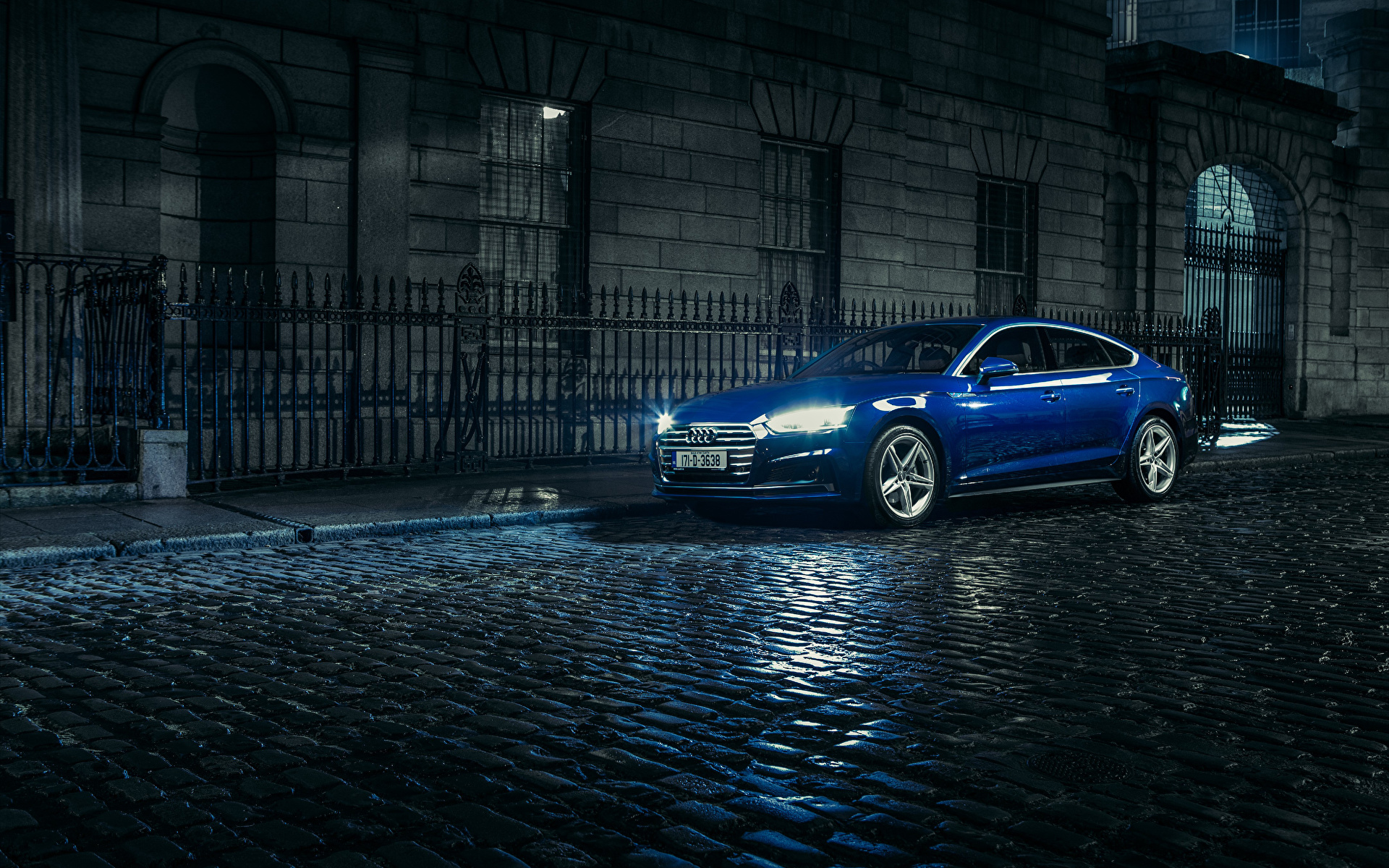This night-time photograph captures an outdoor scene dominated by an intricate brick building in the background. In front of the building stands an ornate black metal fence with pointed pillars and vertical columns, leading to a gated arch doorway. The street in the foreground is cobbled with brick pavers, creating a slightly shiny effect where light glares on it. Centrally positioned in the image, a bright blue, four-door Audi sedan with chrome rims and modern stylish features sits with its headlights on. The car's license plate is visible but the numbers are too small to read.